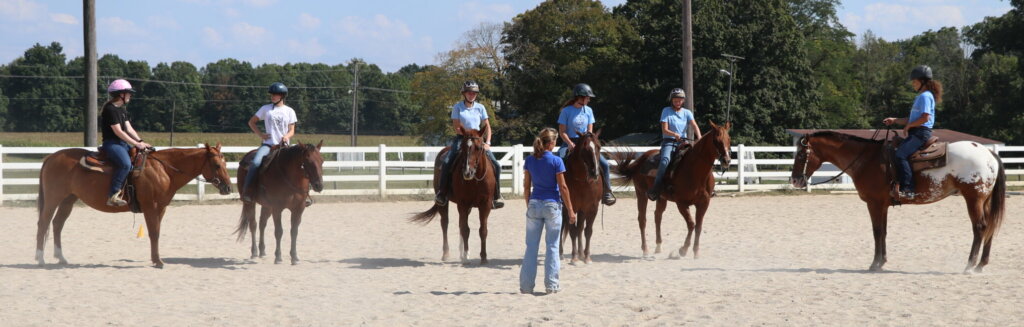In this panoramic image, we see six young riders on brown horses arranged in a semicircle within a sandy corral. The riders are predominantly clad in light blue tops and jeans, all wearing helmets. To the right, four riders wear light blue tops, while on the left, one rider wears a black shirt with a pink helmet, and another wears a white shirt with a black helmet. Central to the composition is a woman with sandy blonde hair in a ponytail, dressed in a blue t-shirt and light denim pants, standing with her back to the camera as she seemingly instructs the group. The corral is encircled by a white wooden fence, beyond which lie open fields, power lines, trees, and a clear blue sky, creating a serene rural backdrop.